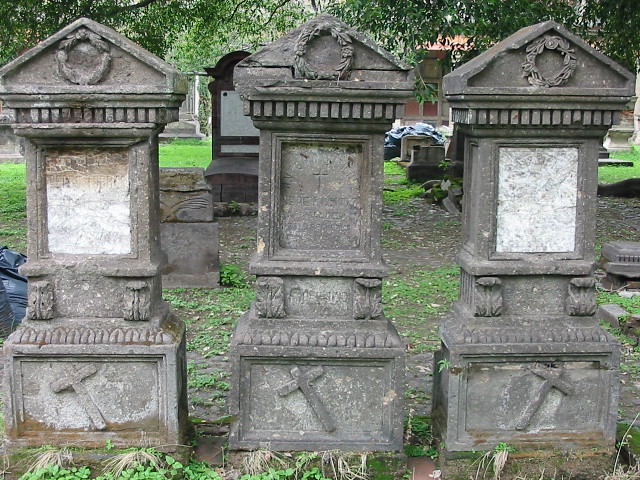In this picture, we see an old cemetery on a bright, sunny day. The primary focus is on three granite gravestones, which are similar in size and shape. Each gravestone features a distinctive design, with a cross at the base: the first two crosses tilt to the left, while the third cross tilts to the right. The monuments have a stylized, house-like top, with engraved wreaths in the shape of laurels in the uppermost section. Below the tops, a rectangular space intended for inscriptions is present—two of these spaces contain faded or damaged images, while the middle one has a carved cross. The gravestones are heavily weathered, with significant chipping and portions missing, making the names unreadable. Surrounding the gravestones are additional, smaller tombstones set in a patch of unkempt greenery. In the background, trees with descending branches provide a shaded canopy. The scene includes discarded garbage bags and tarpaulins near a small granite bench, hinting at neglect. Further back, a building with pink, red, and terracotta details adds depth to the background.